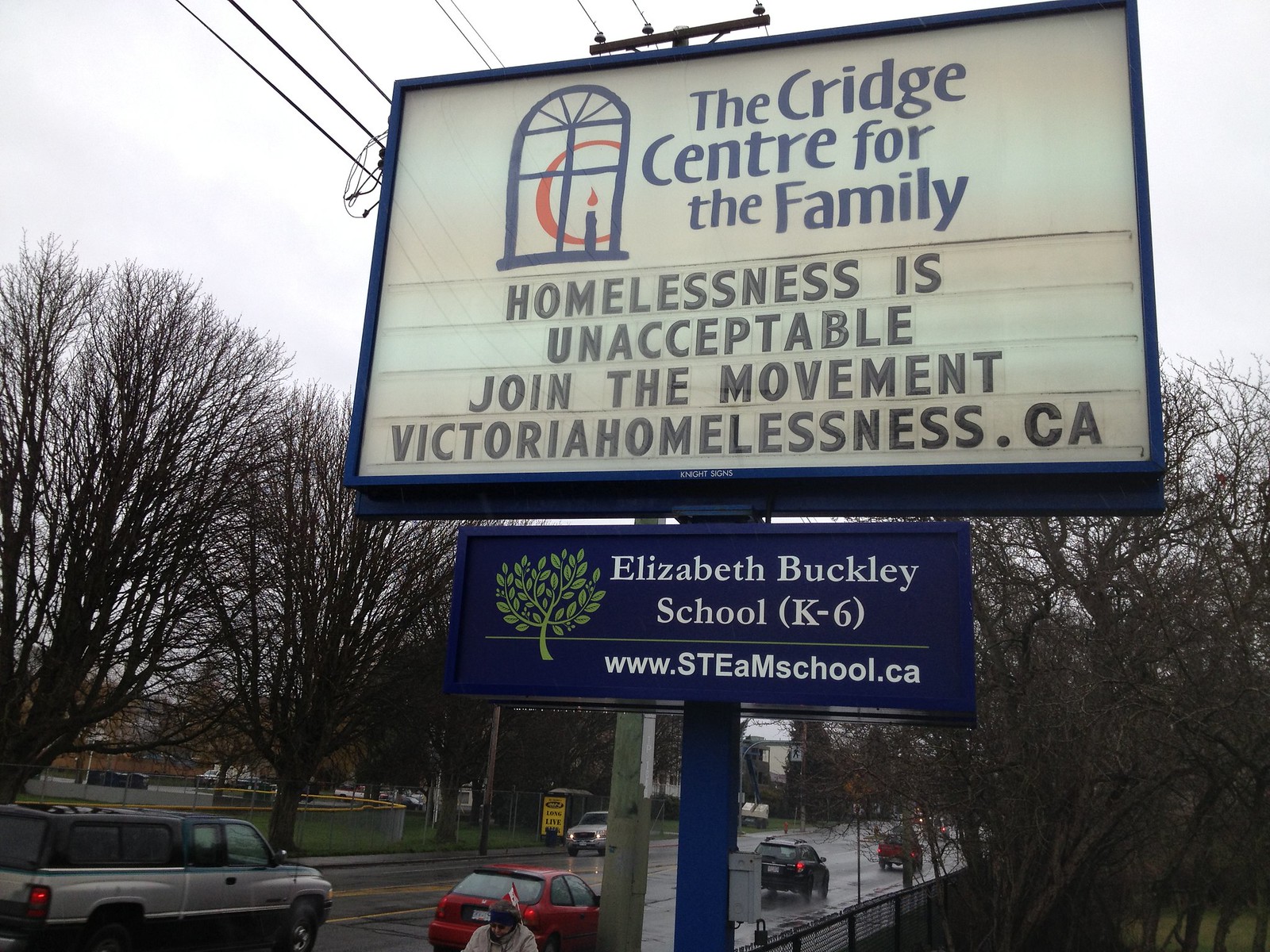This outdoor photograph captures a rainy day scene featuring a prominent sign by a city street. The sign, dominated by a large rectangular blue frame, stands in the foreground and contains two segments. The top segment displays "The Cridge Center for the Family" in black and white, accompanied by a logo of a window with a candle under an arch. Below this, in bold black text, the sign proclaims, "Homelessness is unacceptable, join the movement" followed by the website "victoriahomelessness.ca." The lower portion of the sign features a smaller navy blue board with the text "Elizabeth Buckley School, K-6" and the school's website "www.steamschool.ca". The wet city street beneath the sign is active with traffic, including a silver minivan, two red sedans, a black sedan, and a white car traveling in opposite directions. A woman wearing a hat is seen standing behind one of the red sedans. The background reveals barren trees with thick, dark branches and a telephone pole with wires stretching across the scene, contributing to an atmosphere that suggests late fall or winter.